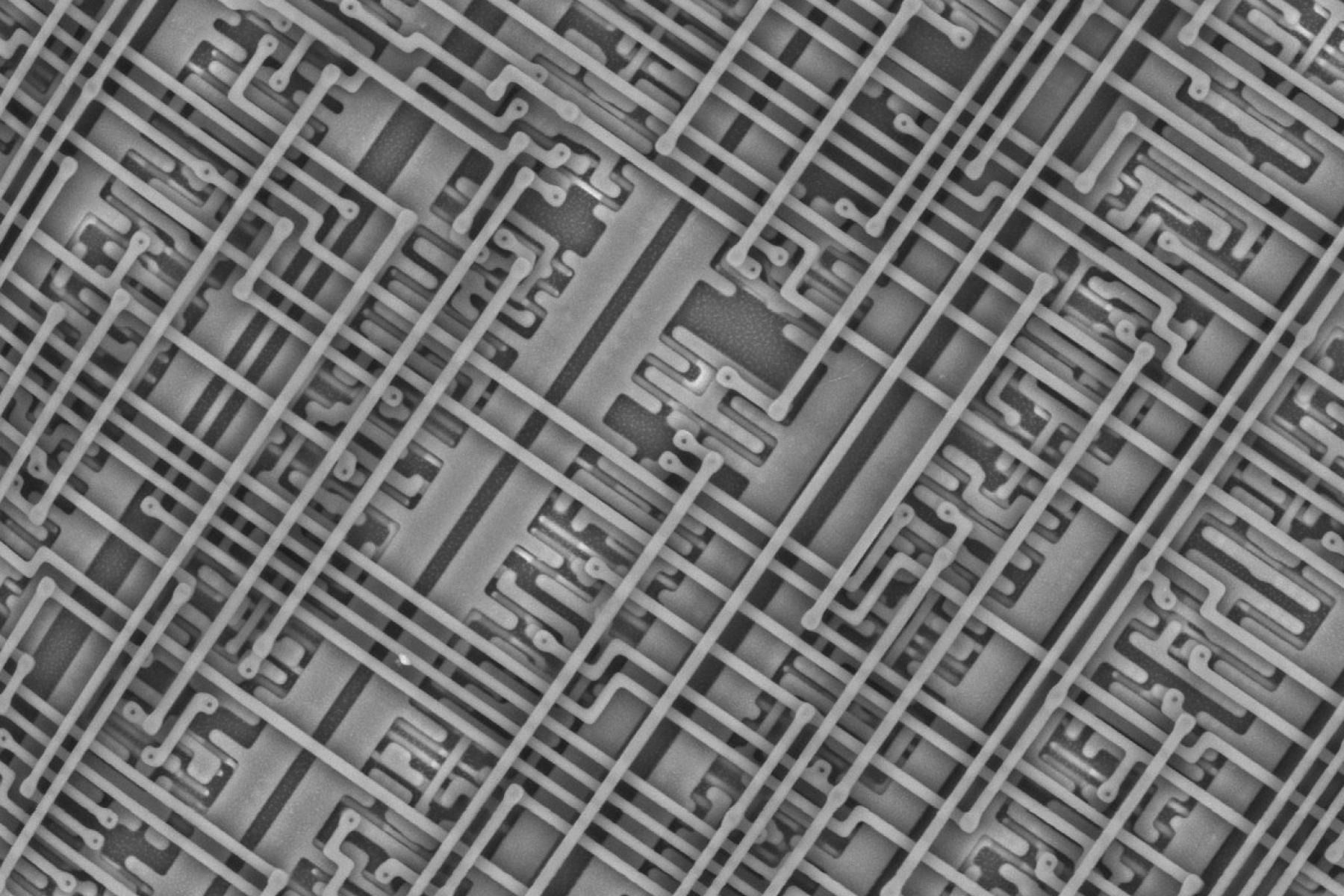The image depicts a detailed, zoomed-in view of a technical, black and white circuit board. Rectangular and square chips are meticulously soldered onto its surface, connected by a network of hair-thin, crisscrossing wires. The wires form intricate patterns, turning at sharp 90-degree angles and weaving across the darker gray background, reminiscent of a maze. The circuit board spans almost the entire frame, highlighting its complexity and obscuring any specific identifying features. This grayscale portrayal removes any color distinctions typically found on such boards, further enhancing the technical, almost instructional feel of the image. The image clarity is high, allowing the precise arrangements of lines and chips to be easily discerned, much like what one might encounter in an instructional manual or video on circuit boards.